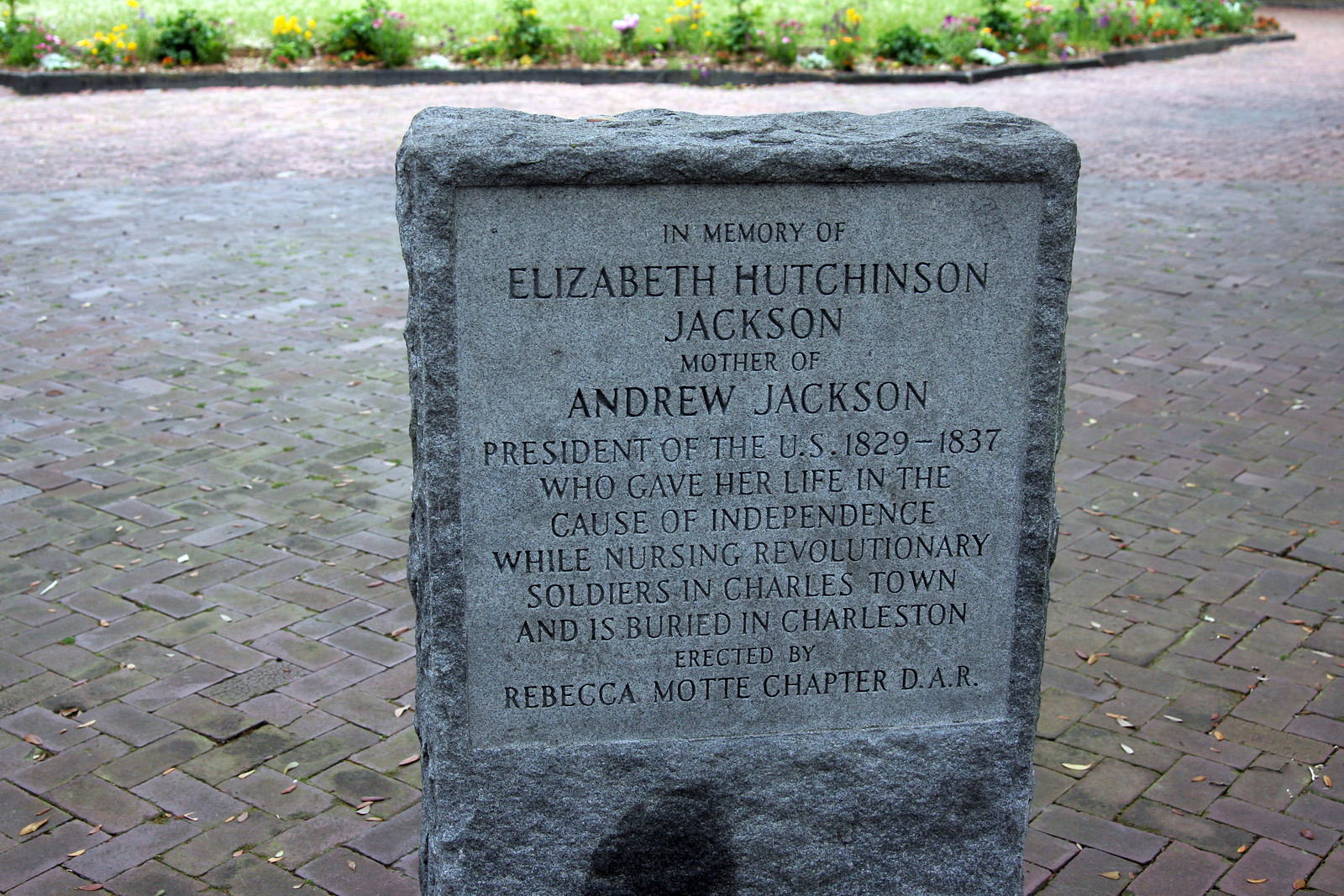In a tranquil courtyard adorned with a bit of a garden, a gray memorial stone stands prominently on a brick-paved path. The stone, resembling a tombstone with a smooth, square engraving on its front face, is dedicated to Elizabeth Hutchinson Jackson, the mother of Andrew Jackson, the 7th President of the United States (1829-1837). The inscription commemorates her sacrifice for the cause of independence, having given her life while nursing revolutionary soldiers in Charlestown, and notes that she is buried in Charleston. This memorial was erected by Rebecca Mott, Chapter D.A.R. Surrounding the stone, small shrubs and vibrant yellow flowers add a touch of nature to the scene, extending to a grassy area in the distance, creating a peaceful park-like setting.